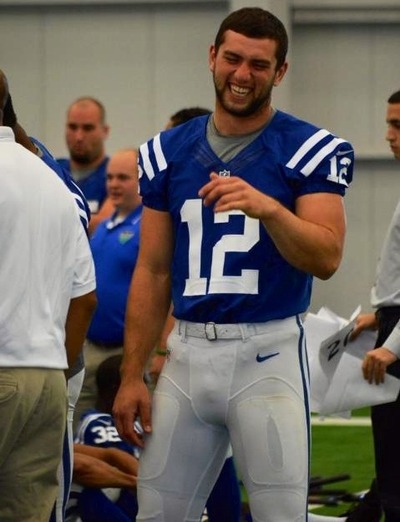The image features an American football player standing in the center, captured from his knees up to his head. He's wearing a blue and white jersey with a large white number 12 on the front and white stripes over his shoulders. A white t-shirt is visible underneath the jersey. His padded pants are primarily white with a blue Nike logo and a blue stripe running down the sides, and he has a white belt. The player has a muscular build, with particularly bulky arms, a dark brown or black beard without a mustache, and short dark brown hair.

He's smiling broadly with his eyes closed, showing his teeth. His right arm hangs down by his side while his left arm is slightly angled upwards and outwards. In the blurred background, there are several people, some wearing attire similar to his and others in different clothing. Notably, a man to his left is in a white t-shirt and brown trousers, while a man on the right, partially visible, is holding papers and wearing a white t-shirt. The bottom of the image shows green grass, with a white wall visible in the background.